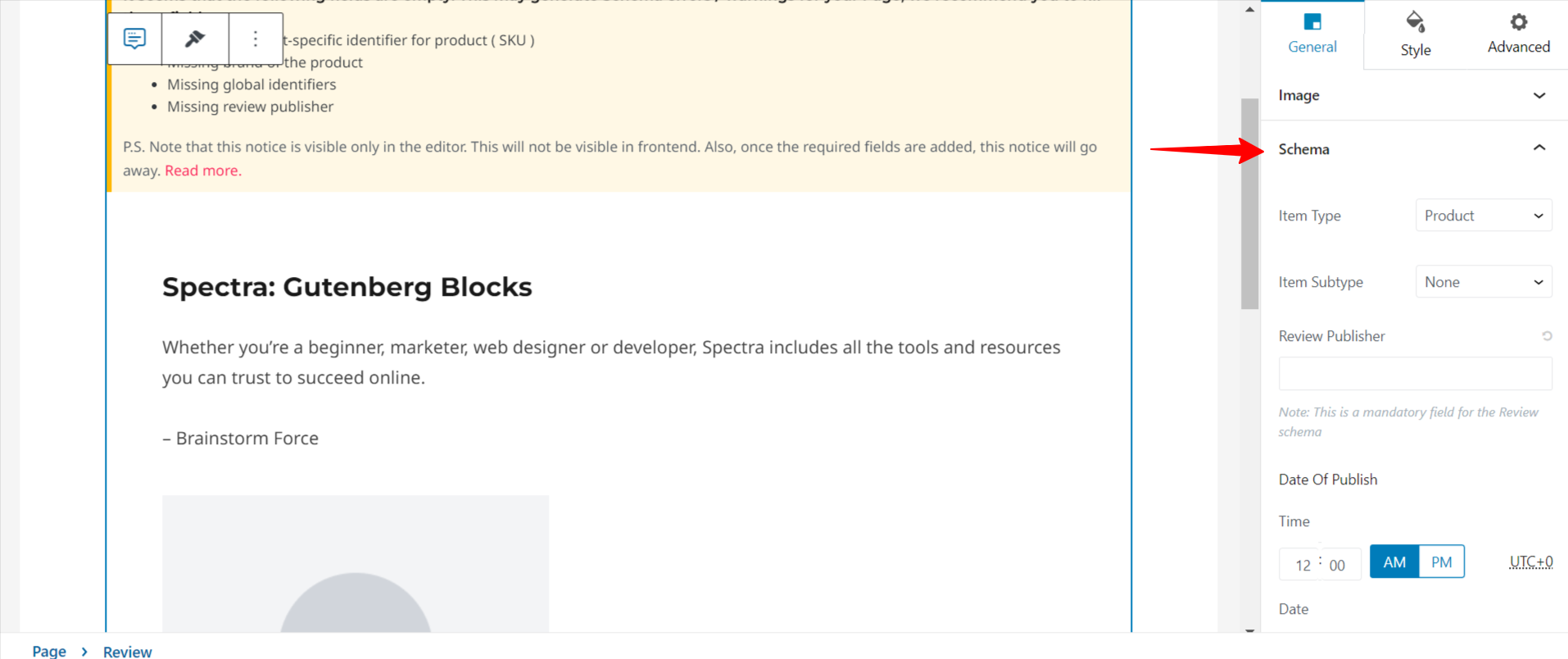**Caption:** 

The screenshot captures the middle portion of a computer screen, scrolled halfway down. At the top, there are three interactive blocks: the first one appears to be for text, the second for painting or drawing, and the third features three dots indicating additional options. These options partially obscure a tan section of a document on the left side. The document contains a message regarding specific identifiers for a product, which highlights missing global identifiers and a missing review publisher. An important PS note at the bottom clarifies that this notice is only visible in the editor mode and won't appear on the front-end. It also mentions that the notice will disappear once the required fields are completed, with an option to "read more" for additional details.

Below this, there's a heading "Spectra: Gutenberg Blocks," with a description explaining that whether you are a beginner, marketer, web designer, or developer, Spectra provides all the tools and resources needed for online success. It mentions the trusted provider "Brainstorm Force" and hints at additional content that isn’t fully visible. 

On the right side of the screen, there are three tabs labeled “General,” “Style,” and “Advanced,” with the “General” tab currently selected. Below this, an image placeholder can be clicked for more options. 

The section displayed under “Schema” on the left includes specific details like item type, item subtype, and review publisher, along with data publishing options that users can choose from.